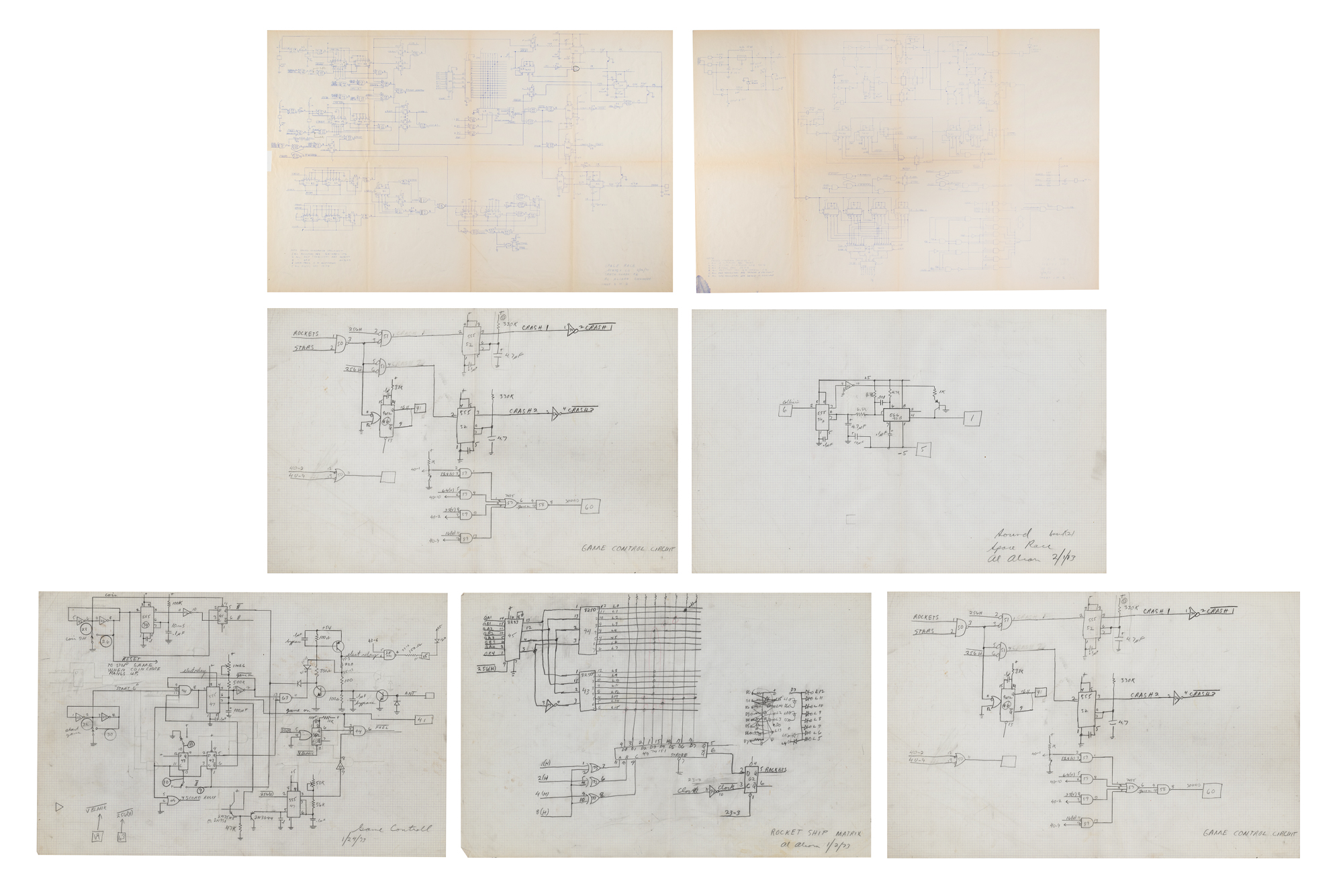The image displays seven rectangular pieces of paper, laid out in a 2-2-3 arrangement, each one featuring what appear to be handwritten electrical schematics. The top row consists of two faint and hard-to-read pieces, with visible fold lines indicating they may have been frequently handled or aged. The second row also contains two pieces of paper with sparser details. The bottom row features three more papers which are more intricate and densely covered with diagrams and calculations. All the pieces seem to be drawn with pencil, marked with various schematics and some text at the bottom, possibly signatures. The background of the image is white, enhancing the worn, beige appearance of the top papers, and the meticulous detail of the line drawings and scribbles across all pieces.